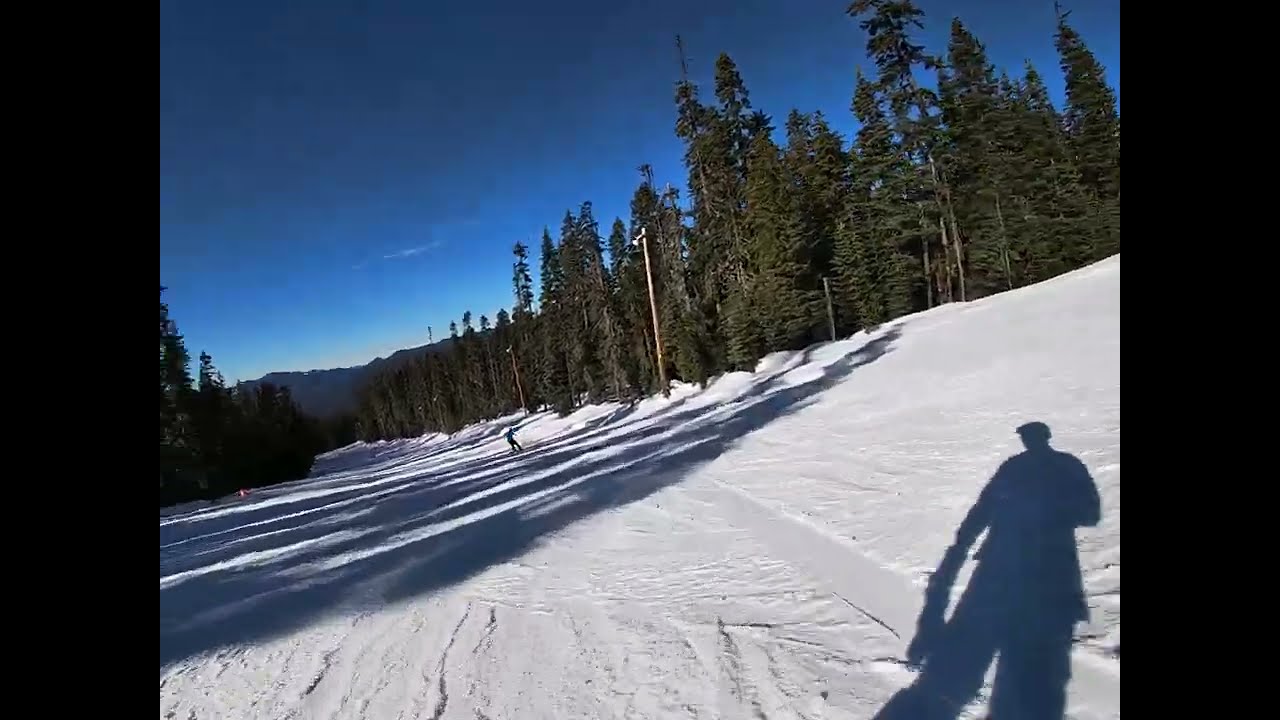In this image, you see the vast, pure white expanse of snow covering the ground, creating a serene and pristine landscape. A huge shadow of a person, likely the photographer, stands prominently on the snow, capturing the viewer’s attention. Surrounding the snow-covered pathway are tall green evergreens or pine trees, casting long shadows across the scene. Among the trees, there are telephone poles with lights, adding a subtle touch of human presence to the natural surroundings. In the distance, a lone snowboarder is visible, gracefully making their way down the slope. Beyond the trees and the pathway, the horizon is marked by the silhouette of brown mountains. Above, the sky is a deep, clear blue, free of clouds, adding to the crisp, tranquil feel of the winter landscape.